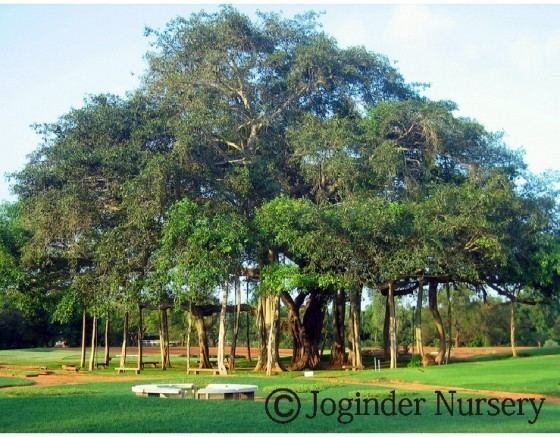The image captures a spectacular outdoor scene featuring a monumental tree that dominates the landscape. The central tree trunk is immensely large, creating the impression of a singular, grand entity. However, there are additional trunks to the left and right, appearing as smaller trees or possibly man-made supports, seamlessly merging their foliage with the main tree to form a unified canopy. Surrounding this magnificent tree are several wooden park benches, strategically placed for visitors to sit and admire the view. A small sandy pathway meanders from the right side of the photo to the left, weaving through lush, verdant grass that covers the foreground. In the background, a serene blue sky adorned with faint white clouds stretches over more distant trees and foliage. A glimpse of a vehicle is visible, partially obscured by the greenery. Notably, the bottom right corner of the image features a copyright symbol along with the text "Joginder Nursery," adding a touch of authenticity to the pastoral scene.